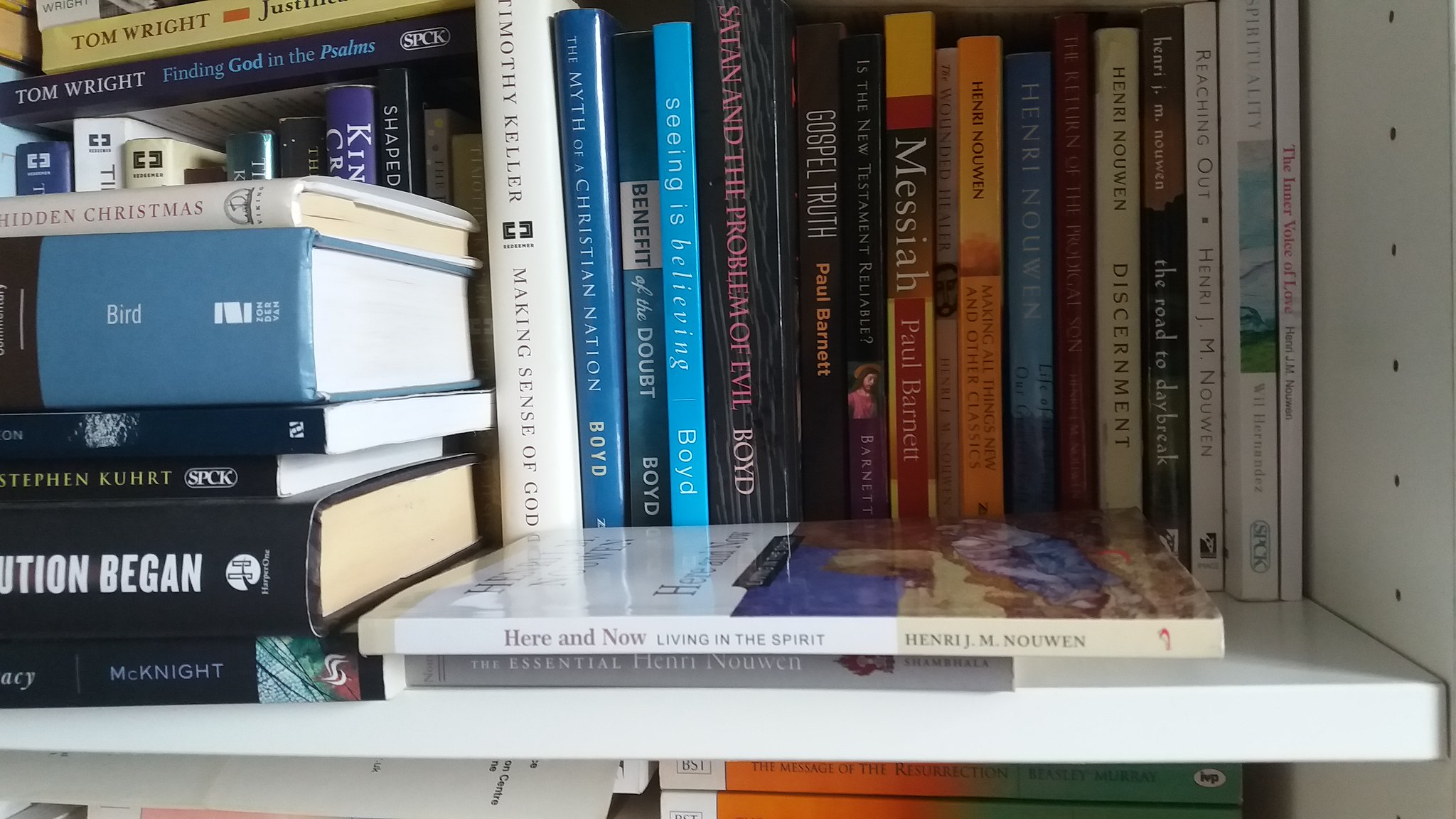This image is an up-close and personal shot of a white bookcase, focusing mainly on two shelves, with books meticulously arranged both vertically and horizontally. The upper part of the image shows vertically placed books with several titles partially visible, suggesting a religious theme. Titles such as "Messiah," "Gospel Truth," "Seeing is Believing," "Here and Now," and "Living in the Spirit" by Henry M. Nouwen are prominently displayed. In front of these vertically placed books, a few are laid horizontally, including one that is partially identifiable as possibly written by Tom Wright, titled "Finding God in..." but the rest is cut off in the frame. The lower shelf contains books stacked horizontally further back on the shelf. Visible titles on the entire bookcase include "Making Sense of God," "The Myth of a Christian Nation," "Benefit of the Doubt," "Satan and the Problem of Evil," "Is the New Testament Relatable," and many more, all by authors whose last names start with the letter B. Approximately 20 books are immediately visible, although the bookcase extends out of the frame, leaving the total number of books uncertain. The composition and selection of books strongly suggest they cater to a readership interested in in-depth religious thought and introspection.